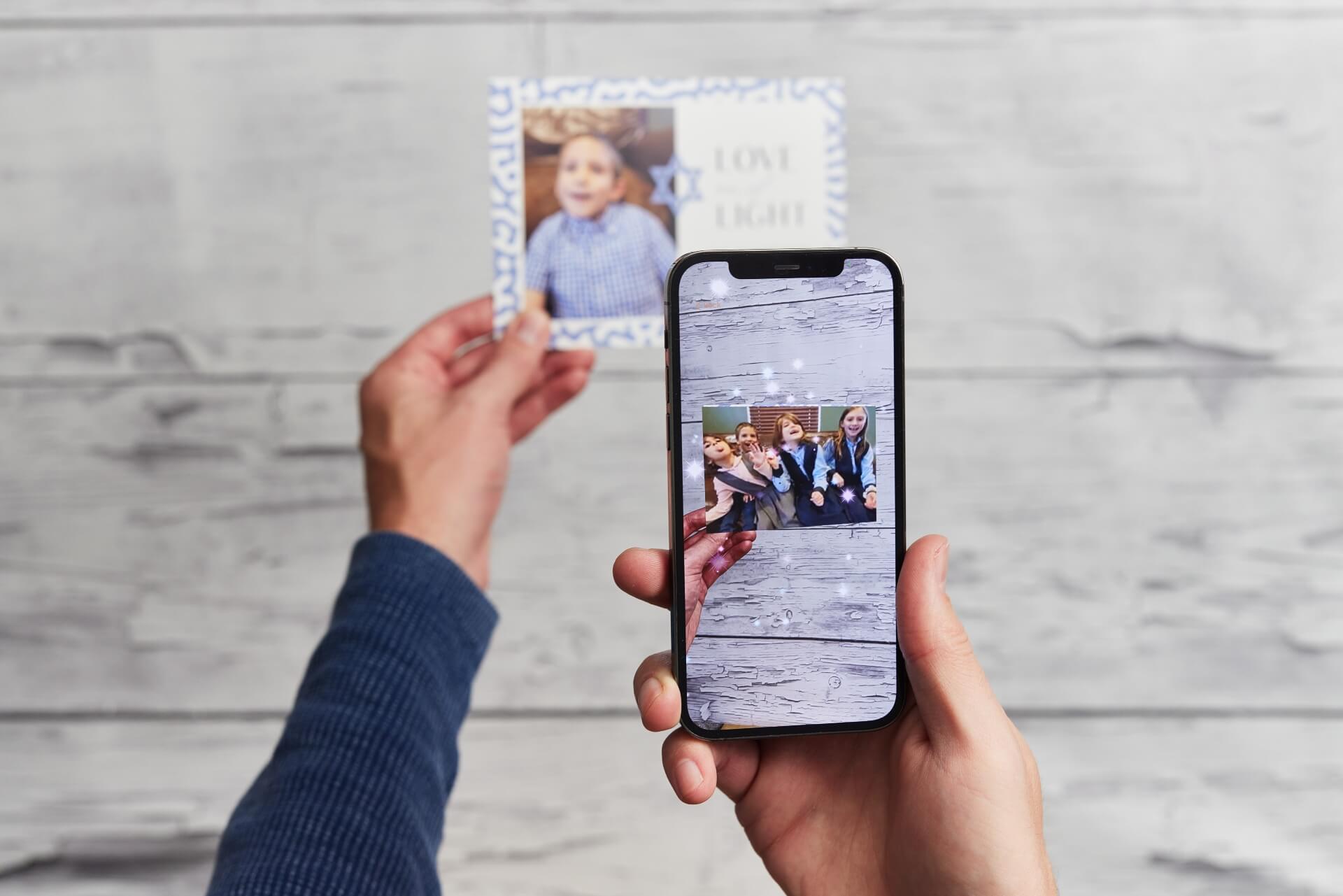In this image, a person is depicted holding a smartphone in their right hand and a photograph in their left hand against a backdrop of a grayish, wooden, panel wall. The smartphone, encased in a black case, shows an image on its screen, which features four children in school uniforms. The boys wear black vests and blue shirts, while the girls don pink vests, all appearing joyful as they sing or dance in front of a red brick building with windows. In their left hand, the individual holds another picture, which resembles a greeting card or postcard. This card showcases a young boy in a button-down blue shirt, with text beside him that reads "Love and Light" along with a Star of David. The dual images – the photo on the phone screen and the postcard-like picture – are unified by the common backdrop of the wooden wall, creating a layered, nostalgic atmosphere.